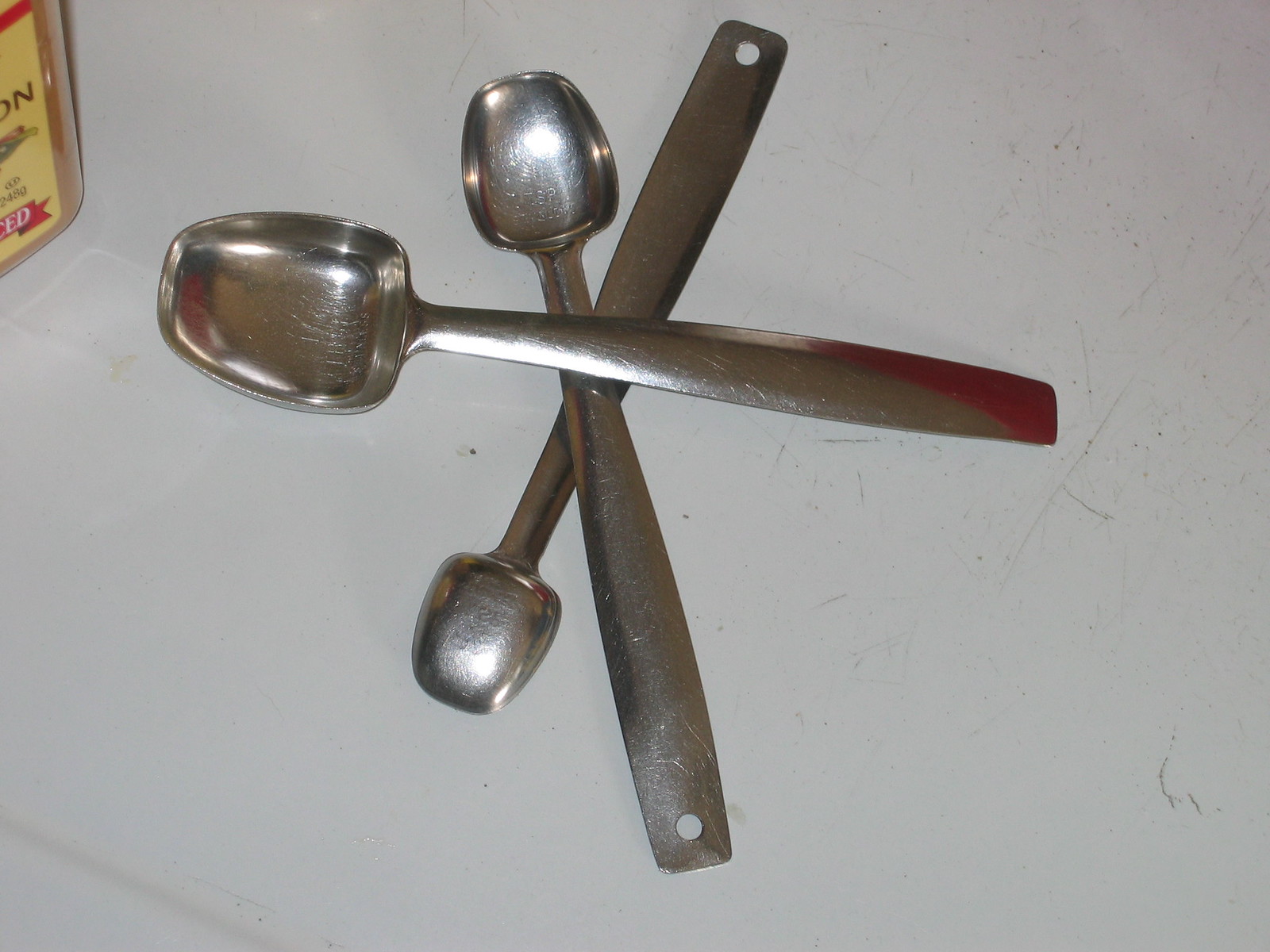In the photo, a white tabletop, marked with years of scratches, serves as the backdrop. In the top left corner, there's a partially visible container, likely holding seasoning, with a yellow label and a hint of a blue ribbon at the bottom. The letters "O" and "N" are barely discernible on this container, which seems to be filled with a brown substance, possibly cinnamon. Centered on the table are three shiny, stainless steel spoons of different sizes, each reflecting light. The largest spoon, oriented horizontally, lies on top of the other two. The medium spoon is positioned diagonally from the upper left to the lower right, and the smallest spoon slants from the bottom left to the upper right. Interestingly, the spoons have a more square-like shape rather than being round, and two of them feature holes at the ends of their handles, suggesting they can be hung up easily. The flash of a camera highlights the metallic surfaces of the spoons, adding a glint to the image.